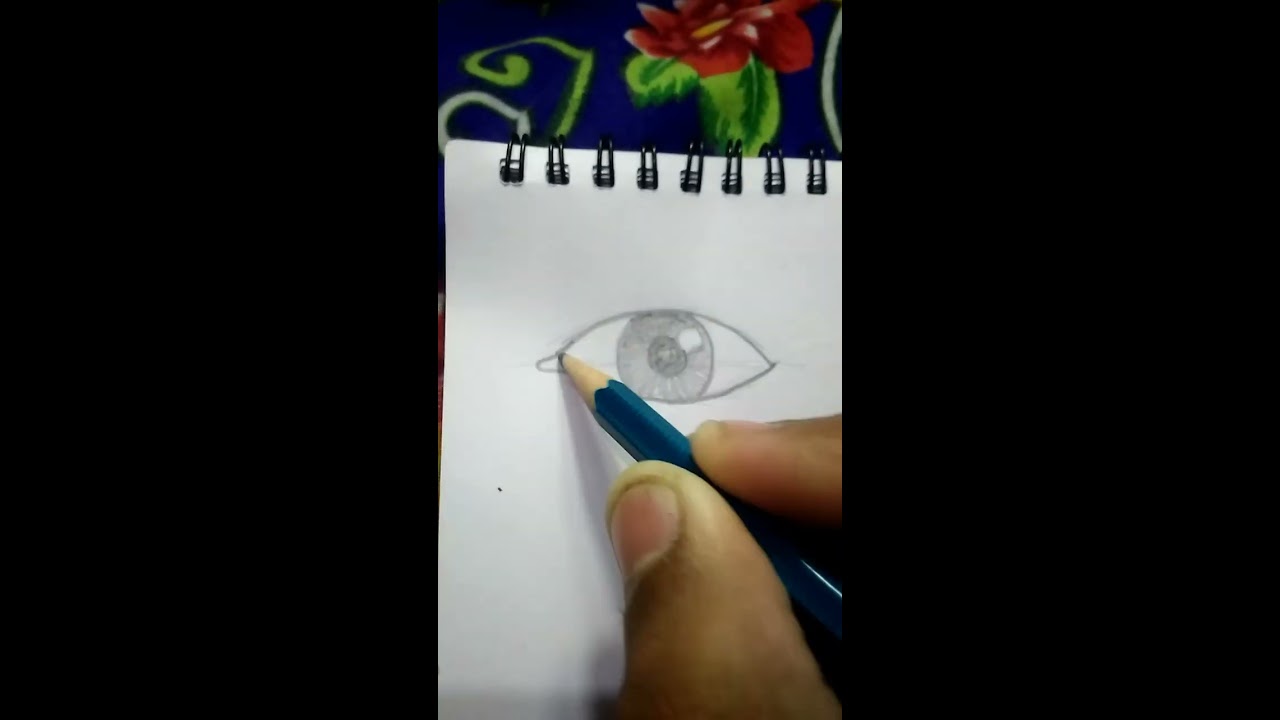This image, likely a still from a video or TikTok, features an individual with darker skin drawing a detailed human eye on a white spiral-bound sketch pad in portrait orientation. The sketch pad, possibly pocket-sized, has black metal spirals at the top and is held against a background filled with a blue floral pattern, complete with green leaves, a red flower with a yellow center, and white lines, reminiscent of either a bed sheet or a curtain. The two fingers visible, the thumb and index finger, have short, possibly dirty nails and grip a light blue pencil, emphasizing the contrast and focus on the drawing. The entire composition is framed by solid black bars on the left and right sides, centering the viewer's attention on the meticulous pencil drawing of the eye in the middle of the frame.